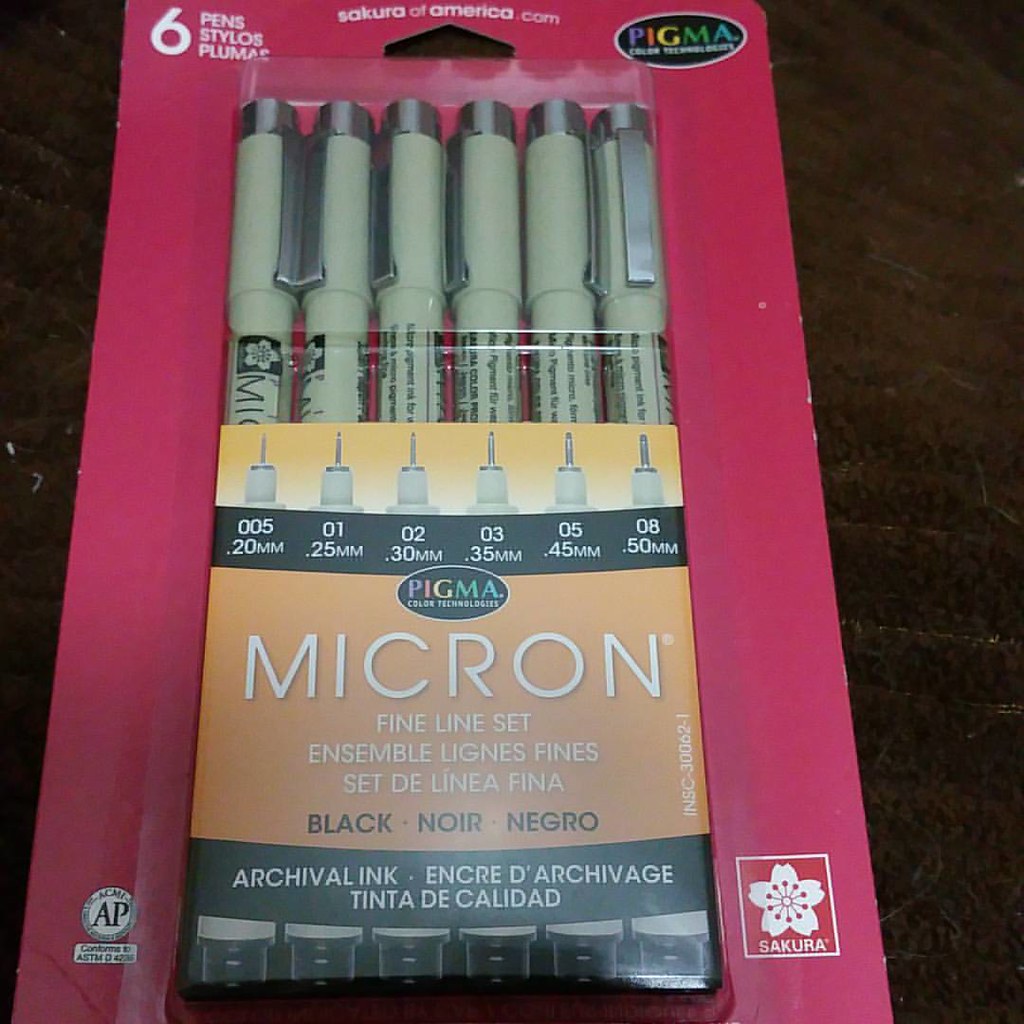The image depicts a portrait-oriented color photograph of a product package containing six Pigma Micron pens, ideal for artistic inking. These pens are housed in a pink and red package with a clear plastic cover that showcases the pens inside. Each pen is beige with silver caps and features black writing indicating their specific sizes. The pens come in varying nib sizes: 0.20mm, 0.25mm, 0.30mm, 0.35mm, 0.45mm, and 0.50mm, suitable for fine line work. The brand logo "Pigma" is displayed in an elliptical black circle with each letter in a different color, located at the top right corner of the packaging. At the top left, it reads "six pens." The label below the pens reads "Micron" in gold with white lettering, followed by "Fine Line Set" in smaller print. The packet further details the pen information in French and Spanish, mentioning "black, noir, negro" to indicate the ink color, and "archival ink" is inscribed in a black curved band with white text at the bottom. The bottom right features a small white flower logo labeled "Sakura." The overall style of the image is realistic, typical of product photography, emphasizing the details and quality of the pens.